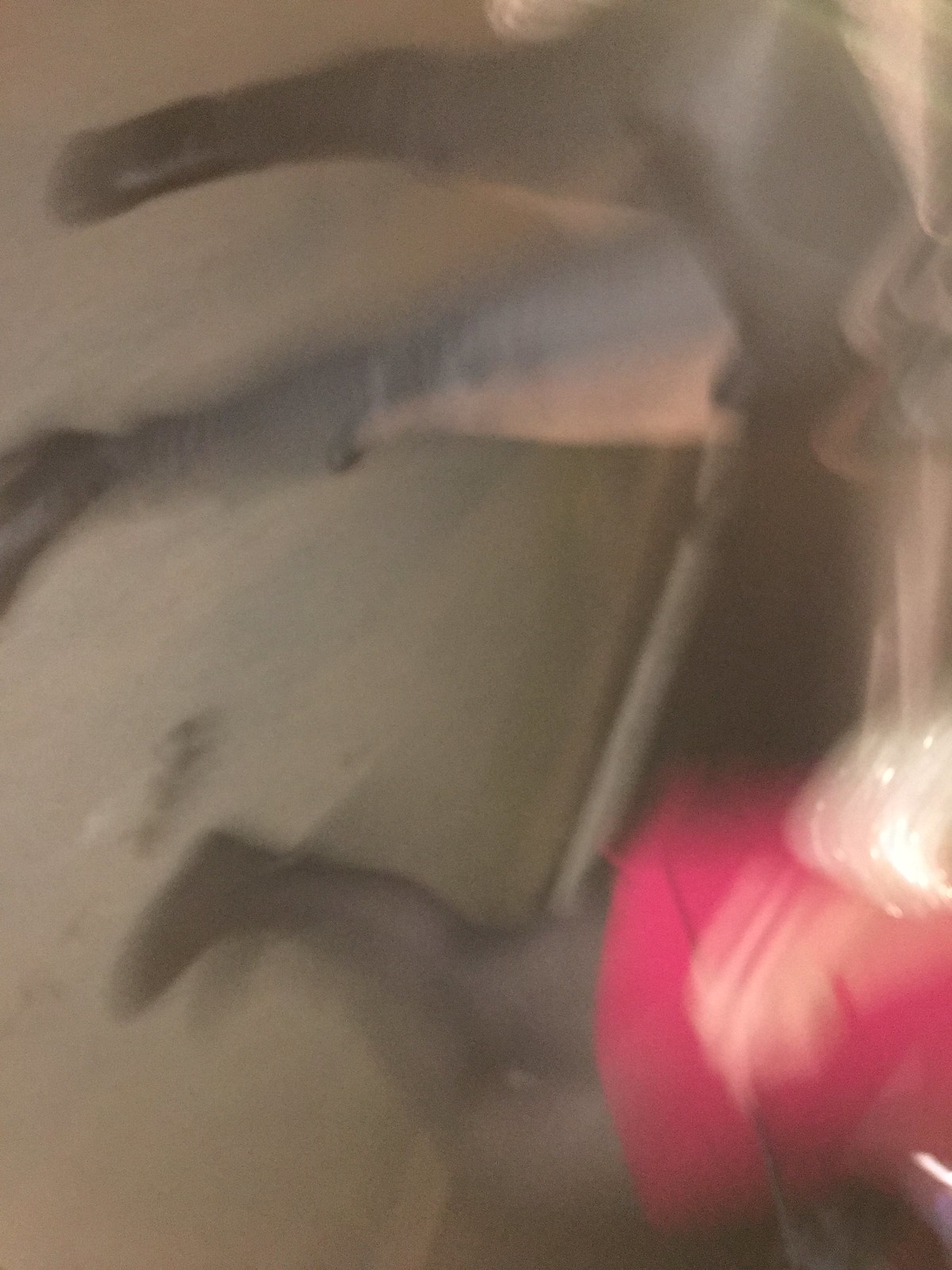This image appears to be an accidental, candid shot taken sideways, resulting in a tall, rectangular photo that is completely blurry. The photo captures the lower halves of two women walking on a stained, dirty sidewalk. Both women are wearing black pantyhose. The woman on the left, slightly shorter than her companion, is dressed in black boots and has a black purse slung around her waist. The woman on the right is wearing black shoes and a red outfit. The blurred nature of the image and its unintended angle give it an abstract quality.